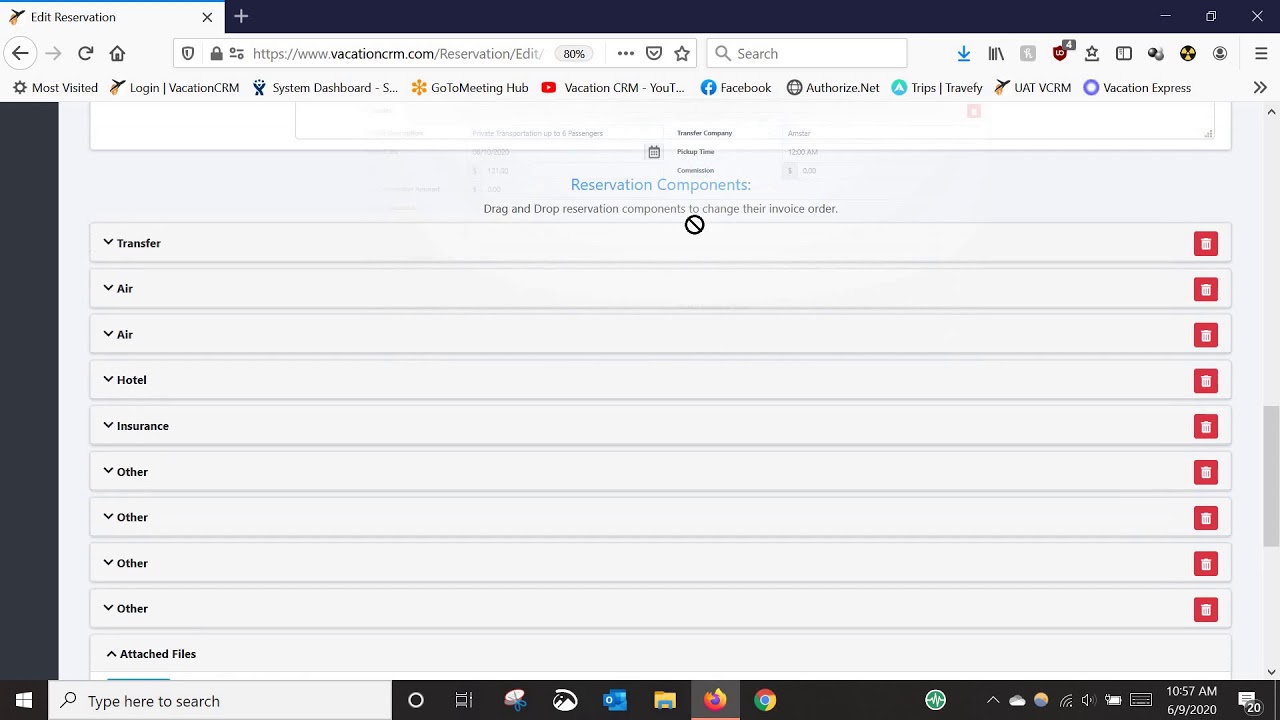Here is a cleaned-up and detailed caption for the image description provided:

---

The image displays a web page from vacationcm.com, specifically designed for editing reservations. The interface features the standard elements of modern web pages, such as navigation tabs, a search bar, and options for downloading content. In addition, there are icons for bookmarking, user profiles, a star for favorites, a refresh button, and arrows for navigating forwards and backwards within the site. A settings wheel is also visible for configuration options.

Prominently featured below the main toolbar is a menu with options like "Most Visited," "Login," "Vacation CRM," "System Dashboard," "Go To Meeting Hub," "Vacation CRM Facebook," "Authorize.net," "Trips," "Travel," "Travelee," "UAT," "VR," "VCRM," and "Vacation Express."

Further down, a section titled "Reservation Components" instructs users to drag and drop various reservation components to adjust their invoice order. The components listed in vertical drop-down boxes include categories such as Transfer, Air, Air, Hotel, Insurance, Other, Other, Other, Other, and Attached Files.

Additionally, there is a search box and a typical browser toolbar interface showing the folder browser for Google and Firefox. The timestamp indicates the current time as 10:57 AM, with the date marked as June 9, 2020. A mini calendar within the interface highlights the 20th of the month.

---

This caption provides a thorough and organized description of the web page's content and layout.